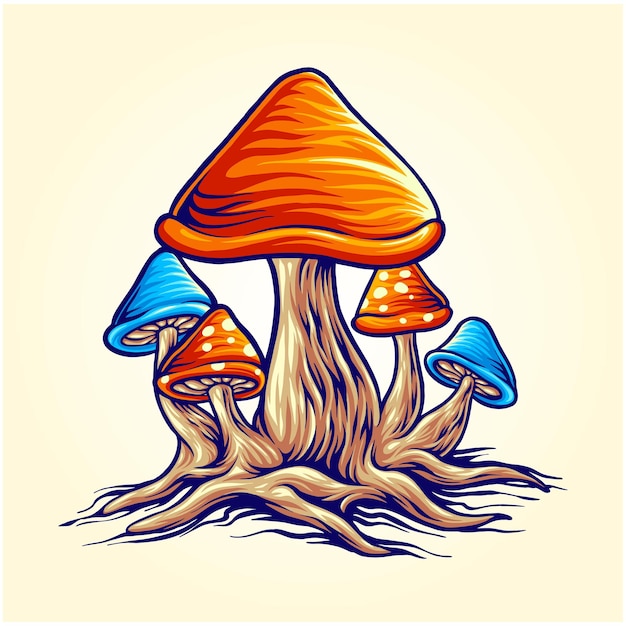The digital artwork depicts a fantastical cluster of five mushrooms against a yellowish white beige background. At the center stands the largest mushroom, with a striking triangular cap adorned with flowing stripes of burnt orange, bright orange, yellow, and white. This central mushroom, characterized by a thick, wooden stalk, connects at the base to the other mushrooms, forming a tree-like structure. The two mushrooms closest to the central stalk are a vivid orange with white polka dots, while the outermost mushrooms display serene blue caps with subtle light blue and whitish lines. Together, the mushrooms exhibit an ombre effect, with colors transitioning from darker shades on the left to lighter hues on the right, adding to the whimsical, imaginative feel of the scene.